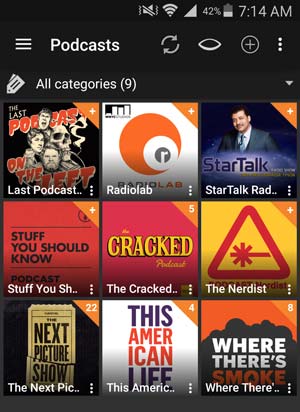This image is a screenshot from a mobile phone displaying a podcast app interface. The background is a dark, charcoal color. At the top right corner of the screen, the status bar shows that the sound is turned off, the Wi-Fi and mobile signals are both at full strength, the battery is at 42%, and the current time is 7:14 AM.

Just below the status bar, the app header is visible in white font, with the word "Podcasts" prominently displayed. To the left of this title, there are three horizontal white lines, which likely open the menu when tapped. On the right side of the title, there are four icons: a refresh icon, a human eye icon, a plus sign, and three vertical white dots (typically indicating additional options or settings).

Further down, in white font, the app displays "All categories, 9," signifying the number of podcasts displayed. Below this, there is a 3x3 grid showing the cover art for nine different podcasts. The top row includes: "Last Podcast on the Left" in the upper left, "Radiolab" in the center, and "StarTalk Radio" on the right. The detailed layout provides a snapshot of the user's podcast selection within a neatly organized interface.